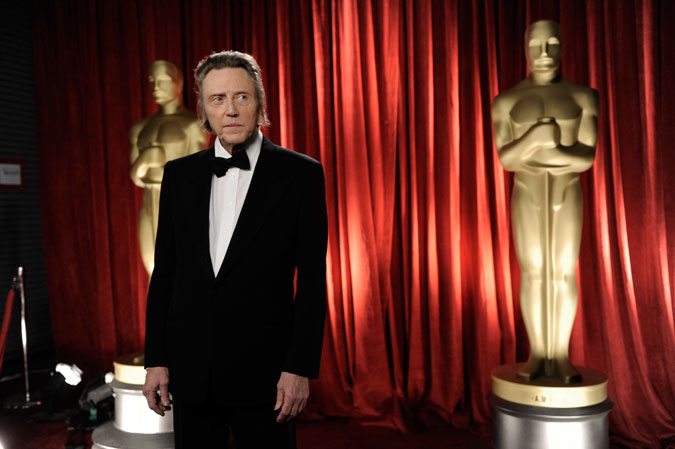In this image, the actor Christopher Walken, a white man likely in his 60s or 70s, stands poised in a black tuxedo with a black bow tie and white dress shirt. His medium-length, slicked-back hair, which is dark at the top and graying at the ends, falls just below his ears. Walken is gazing off to the right with a somewhat droopy facial expression. Positioned slightly forward in the scene, he is framed by two towering, golden statues resembling men holding staffs or swords, each set upon a silver pedestal. Behind Walken and the statues, a long, red, draped curtain bathed in spotlight lighting completes the backdrop. The presence of a red velvet rope on the left suggests a formal event setting, likely an award ceremony.